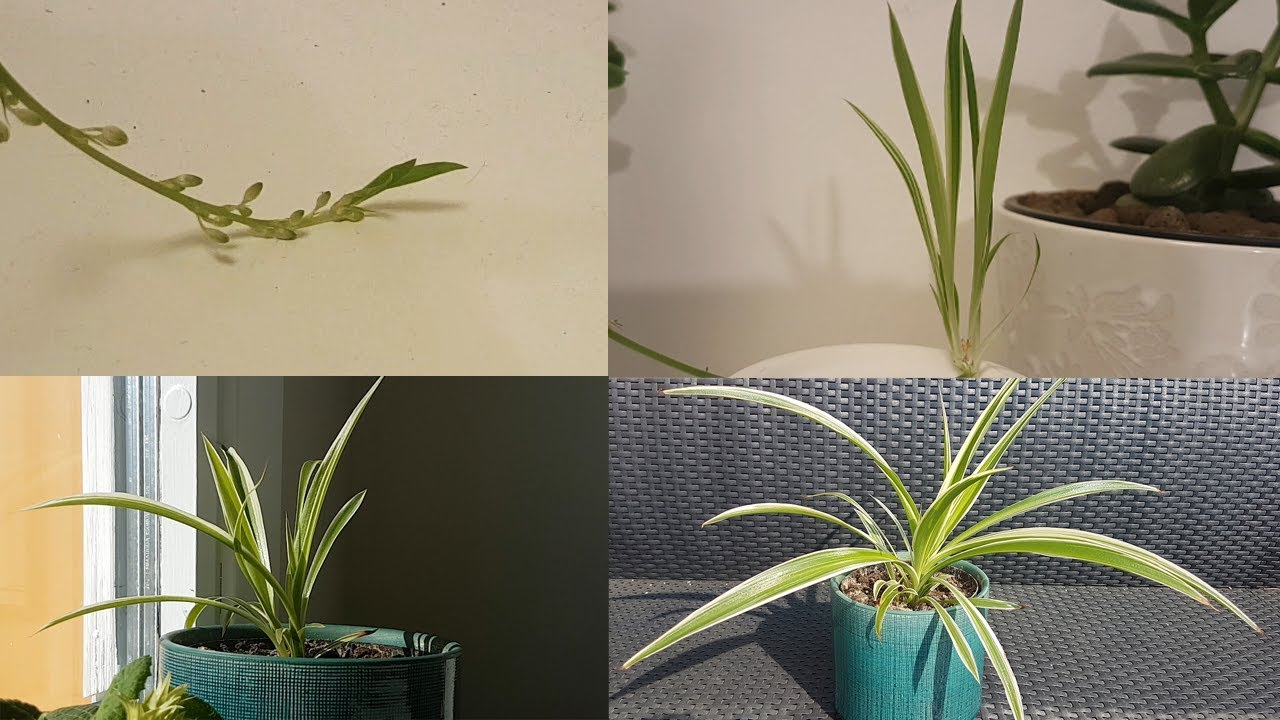The image is a collage composed of four distinct photographs, each showcasing different potted plants. The top left photo, set against an off-white background, features a single curved stem with budding leaves extending from the upper left corner toward the center. To its right, the image shows a dark green plant emerging from a white planter against a white background, with a long leafy plant in the middle foreground. The bottom left picture captures a teal planter on a windowsill casting a shadow, filled with a leafy plant. The final bottom right image displays a more lush and fuller version of a similar leafy plant in the same teal planter, but placed on a wicker surface with a matching backrest. Collectively, the plants featured progress from budding shoots to fuller foliage, including long, palm-frond-shaped leaves, and an additional plant with darker, rounder leaves resembling an elephant's ear in a different blue pot.